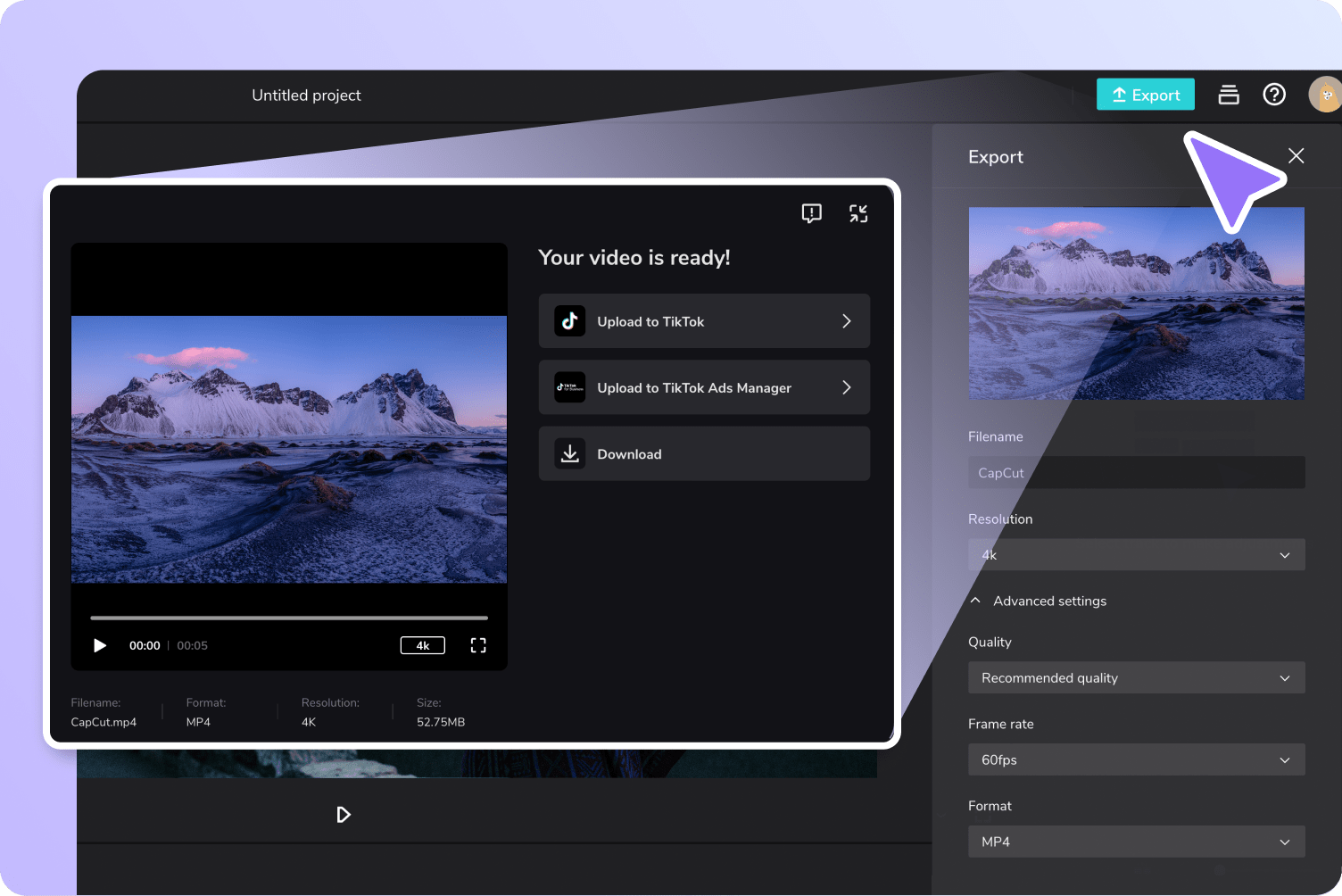The image depicts a light blue background overlaid with a black screen bearing the title "Untitled Project." In the upper right corner, there's a teal button labeled "Export," highlighted by a purple arrow with a white border pointing directly at it. Adjacent to the Export button, several icons are visible, including a circle icon with a question mark.

Beneath the Export button and aligned to the right, there is an "Export" section denoting it has an "X" to close it on the right side. This section features a striking image of an icy, glacier-covered mountain, presumably located in Antarctica or a similar cold region.

Below this image, text details various project settings: 
- File Name: Cap Cut
- Resolution: 4K
- Advanced Settings: Quality
- Recommended Quality
- Frame Rate: 60FPS
- Format: MP4.

Additionally, a pop-up window at the bottom indicates the project status with the message: "Your Video is Ready." It offers options to "Upload to TikTok," "Upload to TikTok Ad Manager," or "Download."